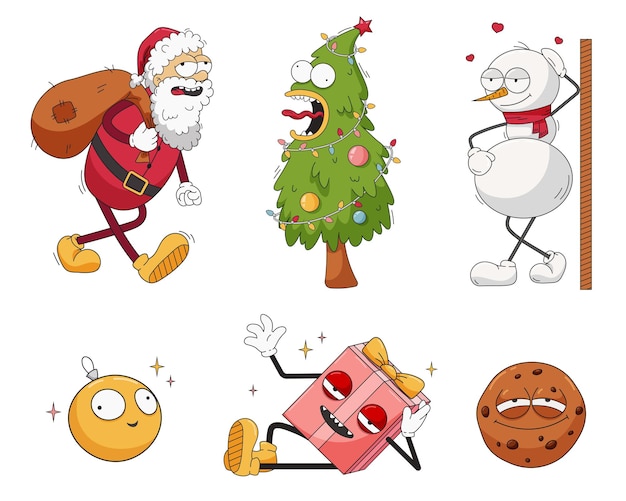On a white background, six whimsical cartoon images are arranged in two rows of three. The top row features a skinny and seemingly exhausted Santa Claus with an open mouth displaying teeth, bulging eyes, and small ears. He wears a red hat, a red Santa suit with a black belt, yellow shoes, and carries a hobo bag over his shoulder. Next to him is an anthropomorphized Christmas tree, adorned with a red star on top and Christmas lights wrapped around it, with a wide-open mouth showing teeth and a thin tongue protruding, and eyes looking in different directions. The last image on the top row shows a snowman (or snow woman), striking a playful pose with one hand on its head and the other on its belly, legs crossed, and three red hearts floating above its head.

In the bottom row, the first image is a yellow Christmas ornament with a smiling face, its eyes slightly askew. The middle image is a pink present with a yellow bow, stick arms and legs, yellow shoes, and is waving while seemingly lounging on the floor with its head propped on one arm. The final image is a chocolate chip cookie with a wide smile, half-open eyes, and an overall relaxed demeanor. Each character is imbued with distinct personality, resembling quirky figures from a cartoon like Rick and Morty.